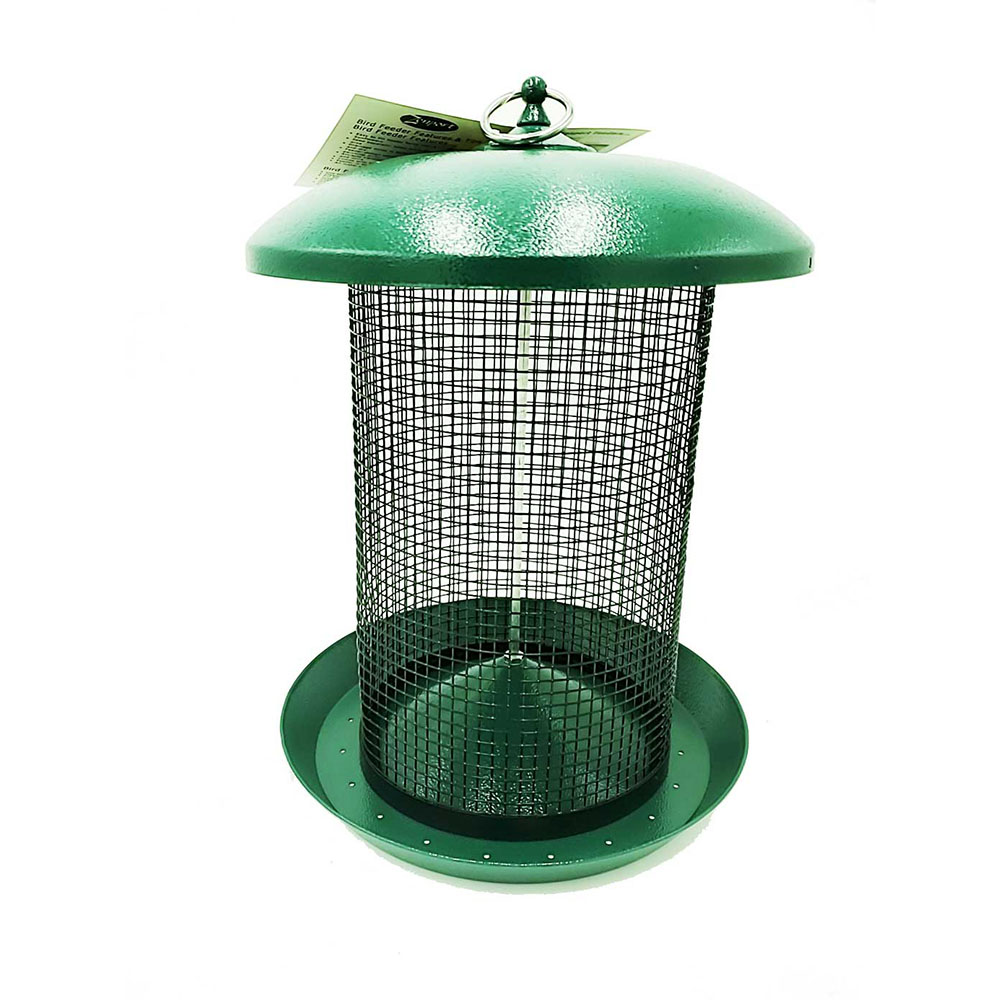The image features a close-up of a brand new bird feeder, designed to resemble a lantern. This feeder boasts an army green color and consists of a green metal disc at both the top and bottom, with a cylindrical square grid metallic netting or cage-like structure in between. The top disc includes a hook for hanging, adorned with a tag that reads "bird feeder" along with additional unreadable text. The bottom disc has a conical section that protrudes upwards into the cylindrical mesh. The overall look is empty, suggesting it is a stock photo for advertising the bird feeder.